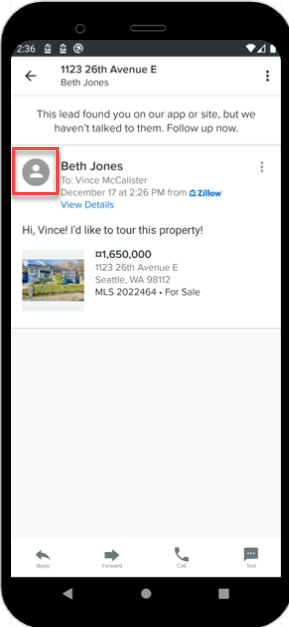The image depicts a black smartphone screen displaying a detailed notification. At the top left, there is a circular icon, followed by a rectangular element slightly lower towards the center. Below this, a gray bar shows various symbols including '2:36', a lock symbol, another lock-like icon, a concentric circle, and a Wi-Fi indicator, along with a triangle with a gray spot and a white element.

The main content begins with a white rectangle featuring an arrow pointing left, labeled "1123 6th Avenue E, Beth Jones". On the right edge of this bar are three vertically aligned dots. Beneath this header, the text reads: "This lead found you on our app, our site, but we haven't talked to them. Follow up now."

A red-outlined rectangle encloses a gray circle with a white person icon, indicating a message from Beth Jones to Vince McAllister, dated December 17th at 2:26 p.m., followed by some blue text that is partially obscured. Directly below is the option "View Details".

The message content reads: "Hi Vince, I'd like to tour this property." Below this request is an image of a house with the text "$560,000" and an address that is hard to decipher, followed by "MLS 202 22 464. For Sale".

At the bottom of the white section, there are icons: a curved arrow pointing left with a word beneath it, a straight arrow pointing right with a word beneath it, a telephone symbol with a word below it, and a speech bubble with a word beneath it.

Lastly, the bottom-most black bar of the phone features navigation buttons: a triangle pointing left (back), a circle (home), and a square (recent apps).